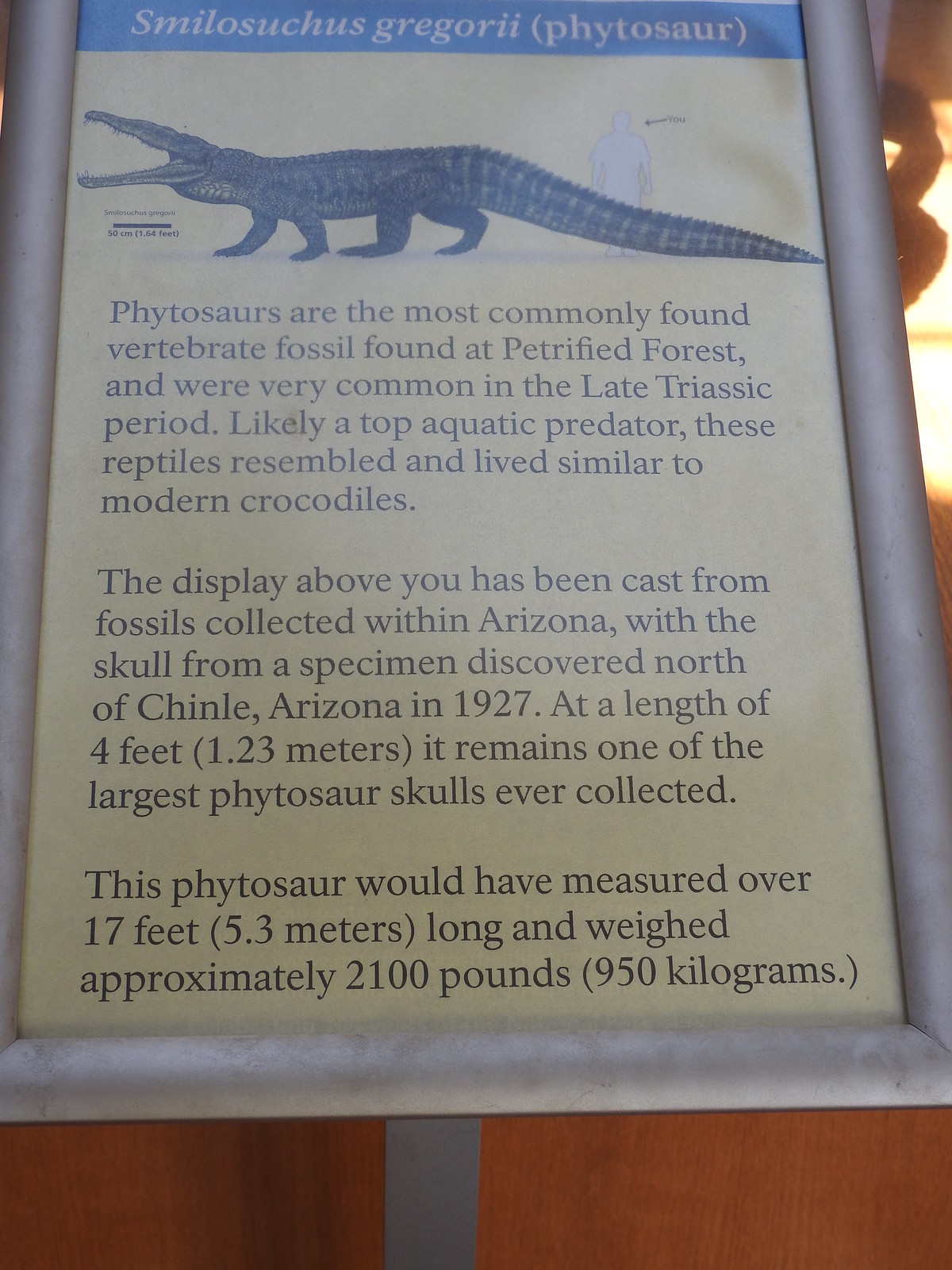This museum exhibit features a detailed display about the Phytosaur species Smilosuchus gregorii. Encased in a silver metal frame with a yellow top banner, the plaque provides extensive information alongside a visual comparison of the Phytosaur's size to that of a human. The illustration showcases the large, ancient reptile, which resembles a modern alligator, towering over an average person. The text explains that Phytosaurs were top aquatic predators during the Late Triassic Period, commonly found as vertebrate fossils in petrified forests. One of the most significant discoveries highlighted on the plaque is a cast of a Phytosaur skull, unearthed north of Chinle, Arizona, in 1927. Measuring over 17 feet in length and weighing approximately 2100 pounds, this 4-foot-long skull remains one of the largest ever found. The exhibit is mounted on a reddish-brown wooden base, suggesting it was photographed in a setting with ample light, likely inside a science museum or zoo.